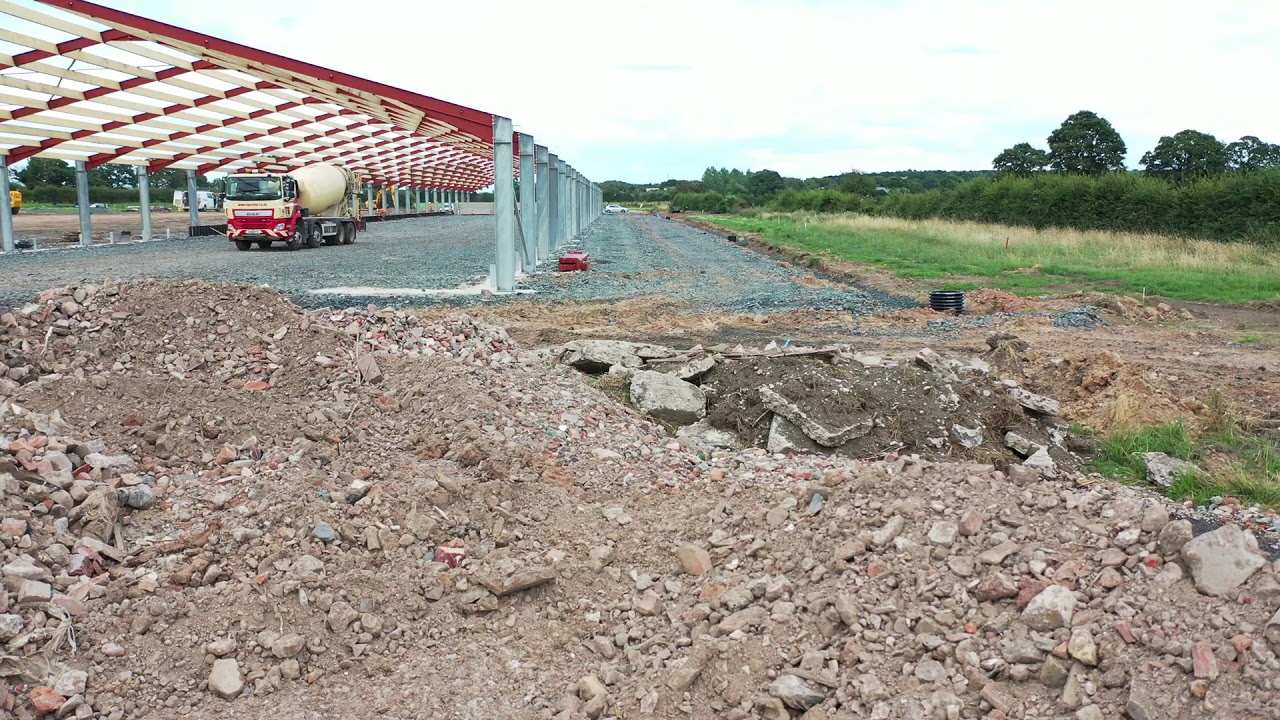This photograph captures a bustling construction site dominated by a vast expanse of brown dirt and broken concrete, dotted with patches of red brick and gray rocks. In the foreground, the terrain is rugged and fragmented, indicating the heavy work in progress. On the left side, a steel framework for a building is being erected, consisting of vertical metal posts and a V-shaped roof structure painted in red and cream colors, suggesting the future shape of a warehouse. In the middle of this skeletal structure stands a cement truck, poised for concrete pouring. Distinguished by its white body and a red stripe, the truck’s rotating mixer is a focal point under the towering framework. To the right side of the image, the chaotic construction environment contrasts with the untouched natural surroundings, featuring tall grass, bushes, and trees seamlessly blending into the background. The image lacks human presence, emphasizing the raw and industrious ambiance of the site.